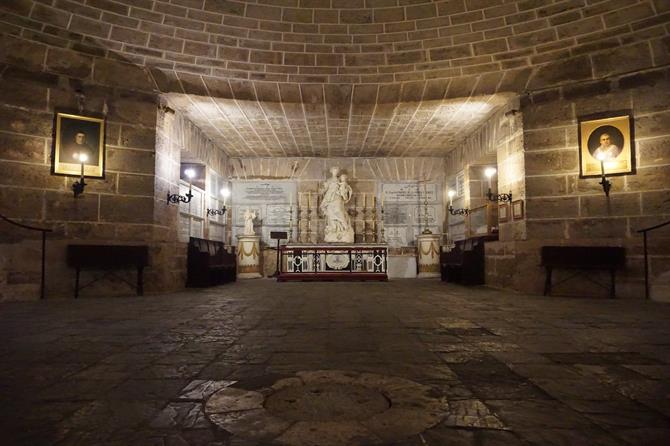The image shows a dimly lit, old brick-walled room with a stone-tiled floor, resembling a cellar or basement. At the far end of the room is a recessed, well-lit section in the brick wall. This section houses a white marble statue of a woman in a long gown holding a baby. The statue is placed on an ornate dark wood chest or table. There are additional details in the surrounding area: on each side of the recessed section, there are inset areas housing different items. On the left-hand side, there's a stand with a smaller marble statue and a picture frame with a black frame and gold matting. On the right-hand side, there's a stand with a golden cross and another picture frame, this time with a circular white matting. Microphone stands and wall sconces are also present on either side, adding to the old-world ambiance of the room.